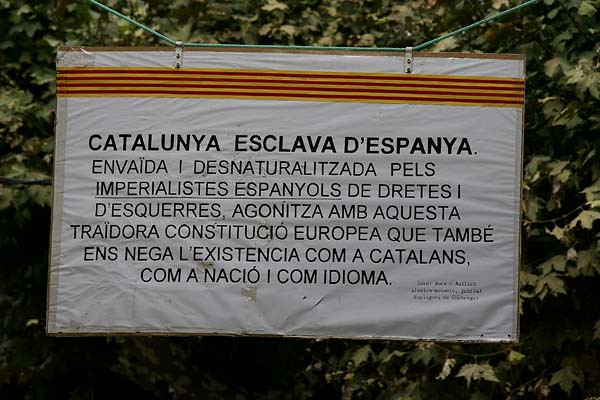The image features a rectangular white sign with black Spanish text prominently displayed, hanging outdoors in a park or wilderness area. The sign is suspended by two metal hooks attached to a green wire or rope. The background is filled with dense, dark green shrubbery and vegetation. At the top of the sign, there is a distinct ribbon-like design with red and yellow stripes reminiscent of a flag. The text begins with the title "Catalonia Esclava de España," followed by several lines of additional Spanish text. The sign's material appears wrinkled, adding texture to its appearance. The scene is brightly lit, indicating it was taken during the day, and the sign is centrally positioned in the image.